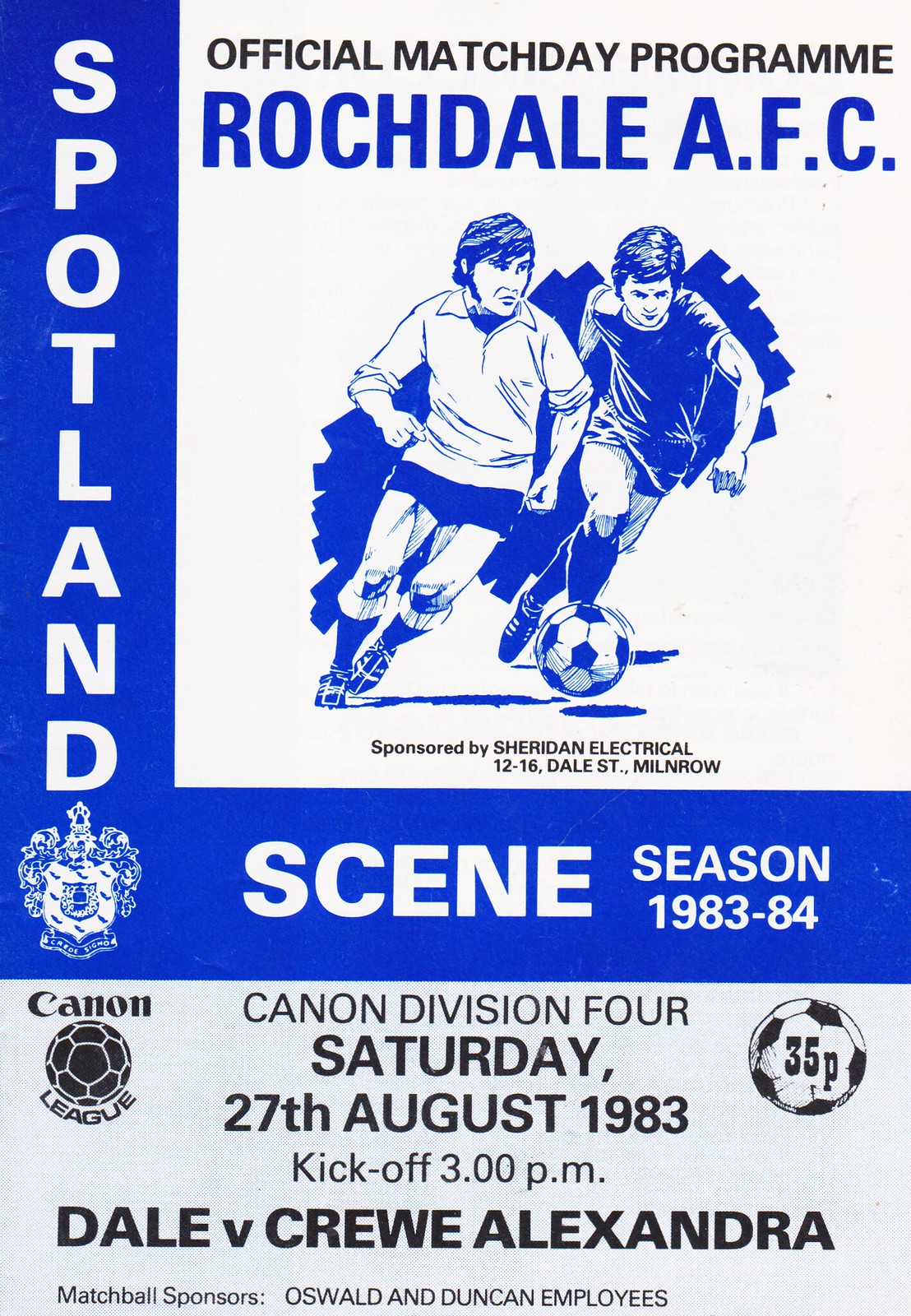This cover of the official match day program for Rochdale AFC features a striking design with blue and white hues. At the top, "Official Match Day Program" is prominently displayed in black text. The title "Rochdale AFC" appears in large blue letters, accompanied by an illustration of two soccer players rushing towards the ball, capturing the dynamic spirit of the game. Vertically aligned on the left is a blue banner with white text that reads "Spotland." Extending horizontally from this banner is the phrase "Scene, Season 1983-84," also in white lettering. A logo representing the football club is set within the blue area. Below the illustration, it mentions that the event is "Sponsored by Sheridan Electrical." Finally, the bottom section of the cover, set in a gray box with black text, provides detailed information about the event, indicating it belongs to the Cannon Division 4 and listing the date, Saturday, 27 August 1983, the kickoff time at 3 p.m., and the teams involved: Dale and Crewe Alexandra.